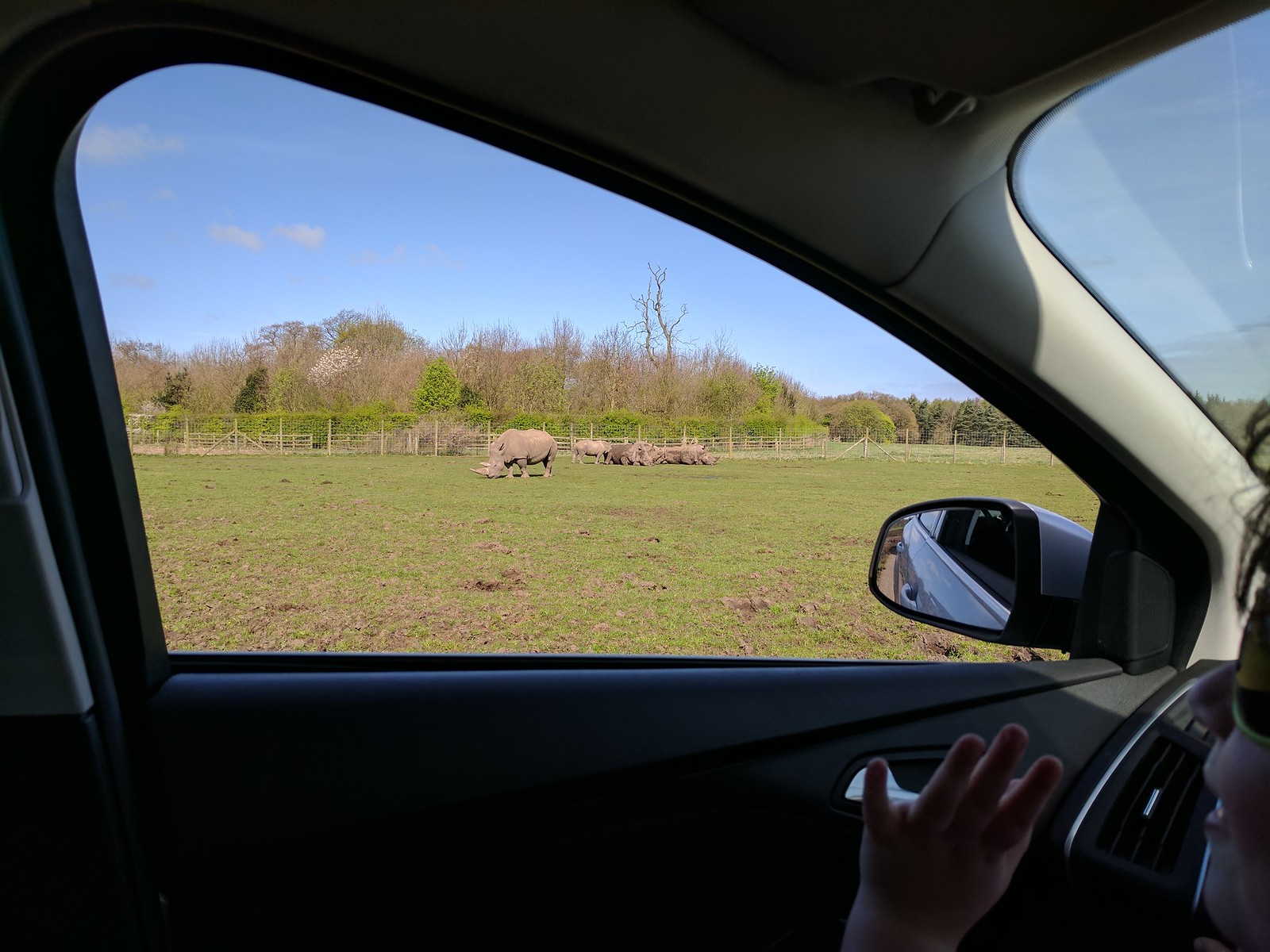The image showcases a picturesque outdoor scene viewed from the inside of a car. From the driver's side window, you can see a smiling little boy with his hands raised as if waving. The background reveals a vibrant field where several rhinoceroses roam. The rhinoceroses are primarily a dusty brownish-gray color, with the one closest to the front gazing downward, its prominent horn in clear view. Behind this one, other rhinoceroses are clustered together, some appearing to lounge while others stand facing different directions. The scenery includes patches of green grass interspersed with brown spots, as well as brown-weeded and lush green trees, along with some bare branches. Beyond the animals and vegetation, a beige wooden fence outlines the yard. Above, the sky is a medium blue dotted with small, dispersed white clouds, adding to the serene landscape.